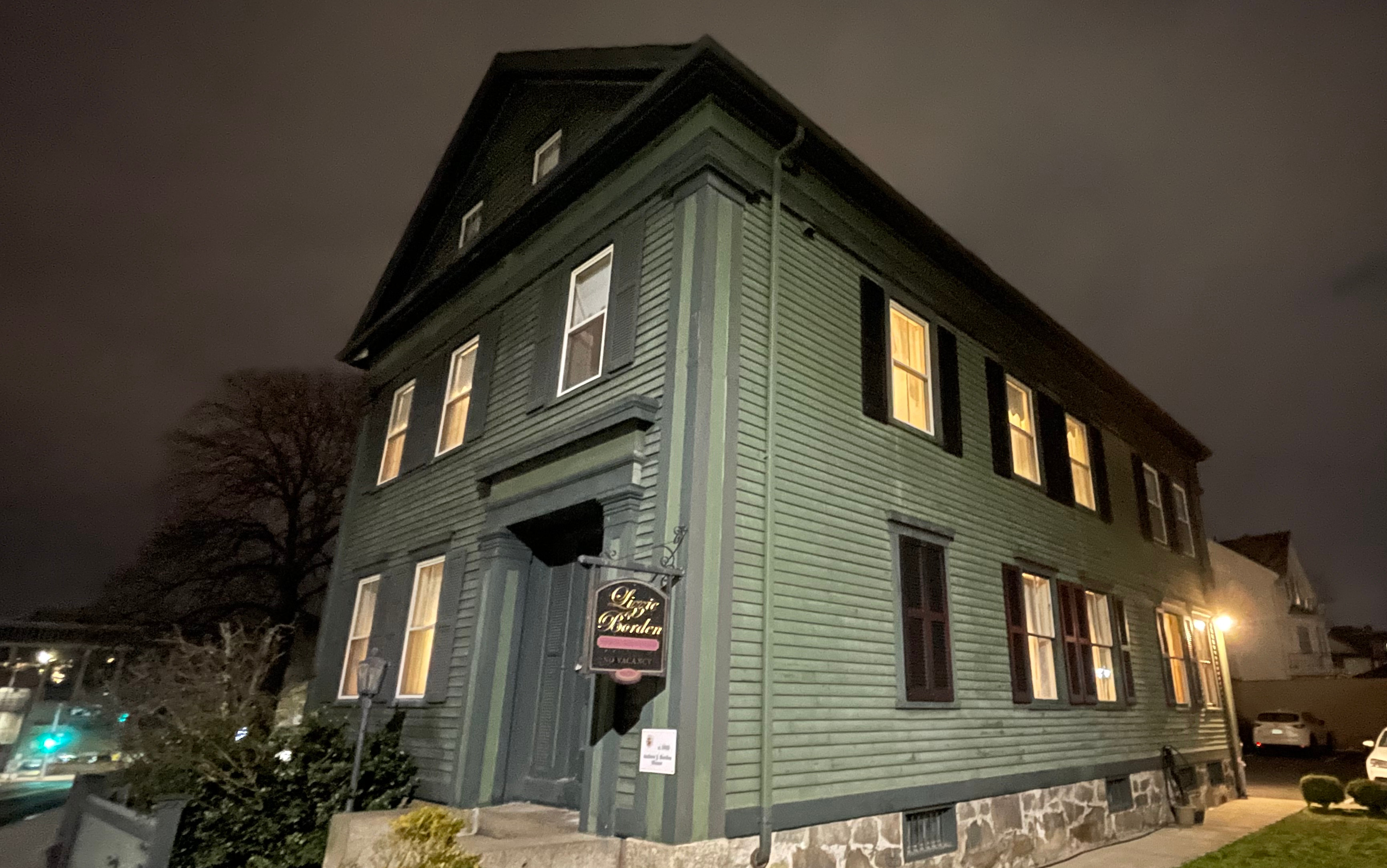The image depicts a historic two-story building situated at night, likely serving as an inn or bed and breakfast given the prominent signage indicating "Lizzie Borden" in gold-colored font, with "No Vacancy" underneath. The building is clad in green-hued hardy board siding, complemented by dark gray/black shutters and white window frames. It rests on a substantial stone foundation, possibly made from limestone or gray sandstone, adding a touch of antiquity to the structure. The roof features attic windows, hinting at additional space above. Soft lighting illuminates the building, and a streetlight near the front porch remains unlit. The surroundings include a well-lit parking lot, a neatly paved sidewalk leading to the green-painted front door, and hints of a swimming pool in the background. Dark, stormy clouds fill the night sky, casting an eerie ambiance over the scene.